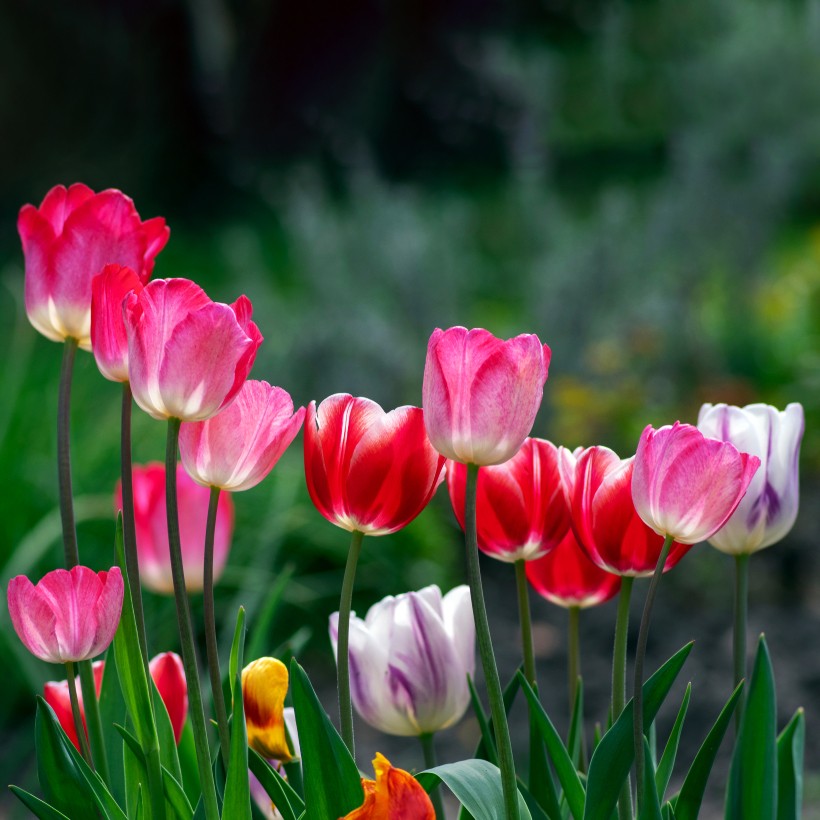This outdoor photograph captures a vibrant and colorful display of blooming tulips arranged primarily in a horizontal row across the center of a square-shaped frame. The main row, located around the middle of the image, features 11 tulips in various shades of pink, ranging from pastel hues to dark, almost red tones. The most striking among them is the rightmost tulip, which stands out with its white petals accented by subtle purple streaks. 

In the lower left corner, partially hidden by green leaves and the tall, straight stems of the tulips, additional blooms can be spotted. These include tulips in pink, white with purple accents, and even a couple that are yellow and orange. The petals of the tulips are clearly defined, upright, and distinctly U-shaped.

The background of the photograph is softly blurred, composed of different shades of green, suggesting outdoor foliage. The very far background fades to black, contrasting smoothly against the vivid colors of the flowers. Overall, the tulips are brightly lit, suggesting a sunny day, and their vibrant colors draw the viewer's attention, creating a lively and picturesque scene.